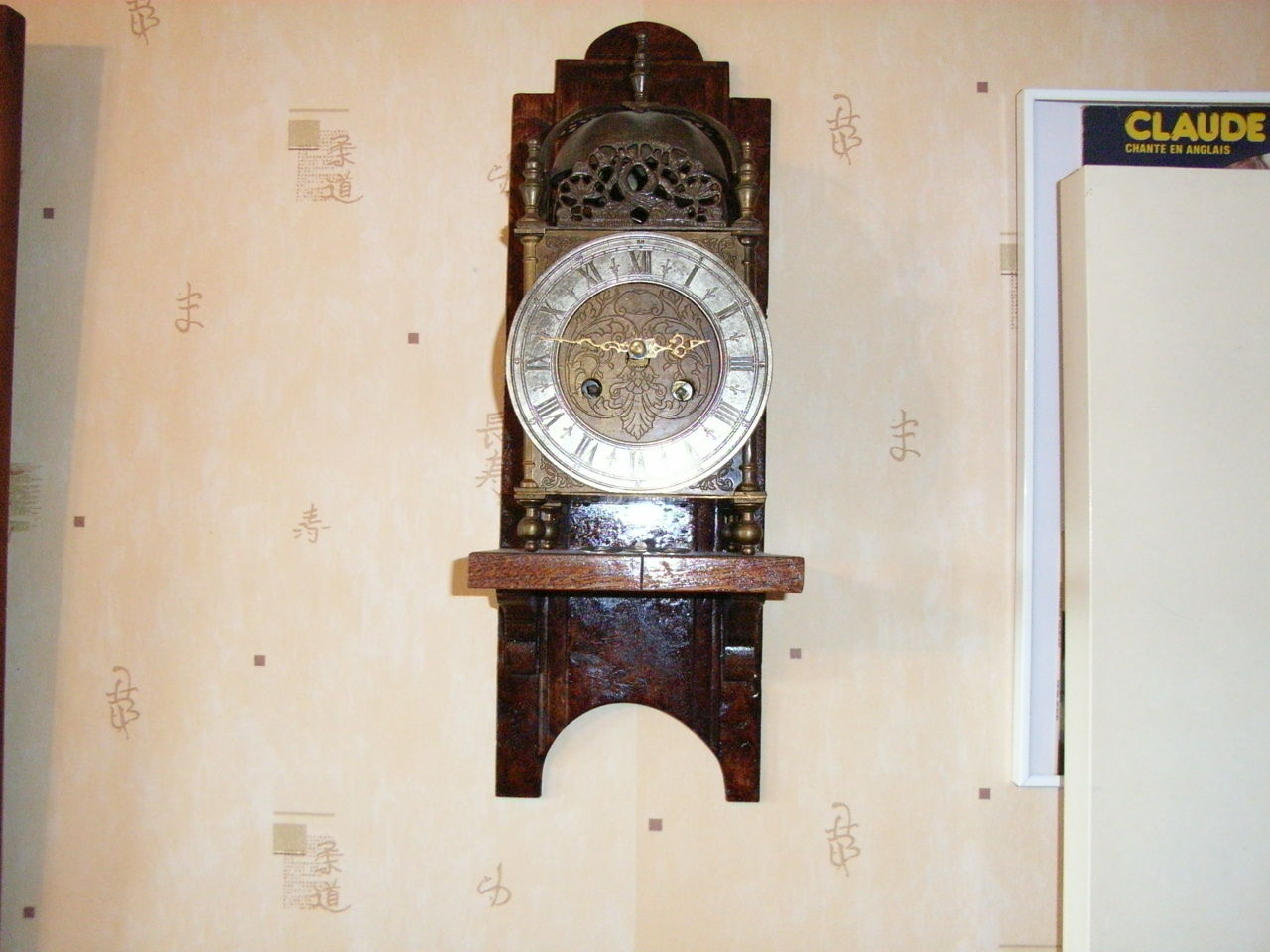This image features a vintage wooden clock, prominently hanging on a tan wall adorned with elegant Asian lettering. The clock's face, made of what appears to be metal or silver, displays the time as 2:47, with ornate gold hands—one short hand slightly past the two and a longer hand a bit beyond the nine. The dial is marked by Roman numerals, adding to its antique charm. The clock's wooden casing exhibits intricate craftsmanship, with a hand-carved, beautifully stained surface. The top of the clock is particularly notable for its detailed floral-like wooden carvings. To the right of the clock, there is a white door with a small cutout above it, displaying the name "Claude."